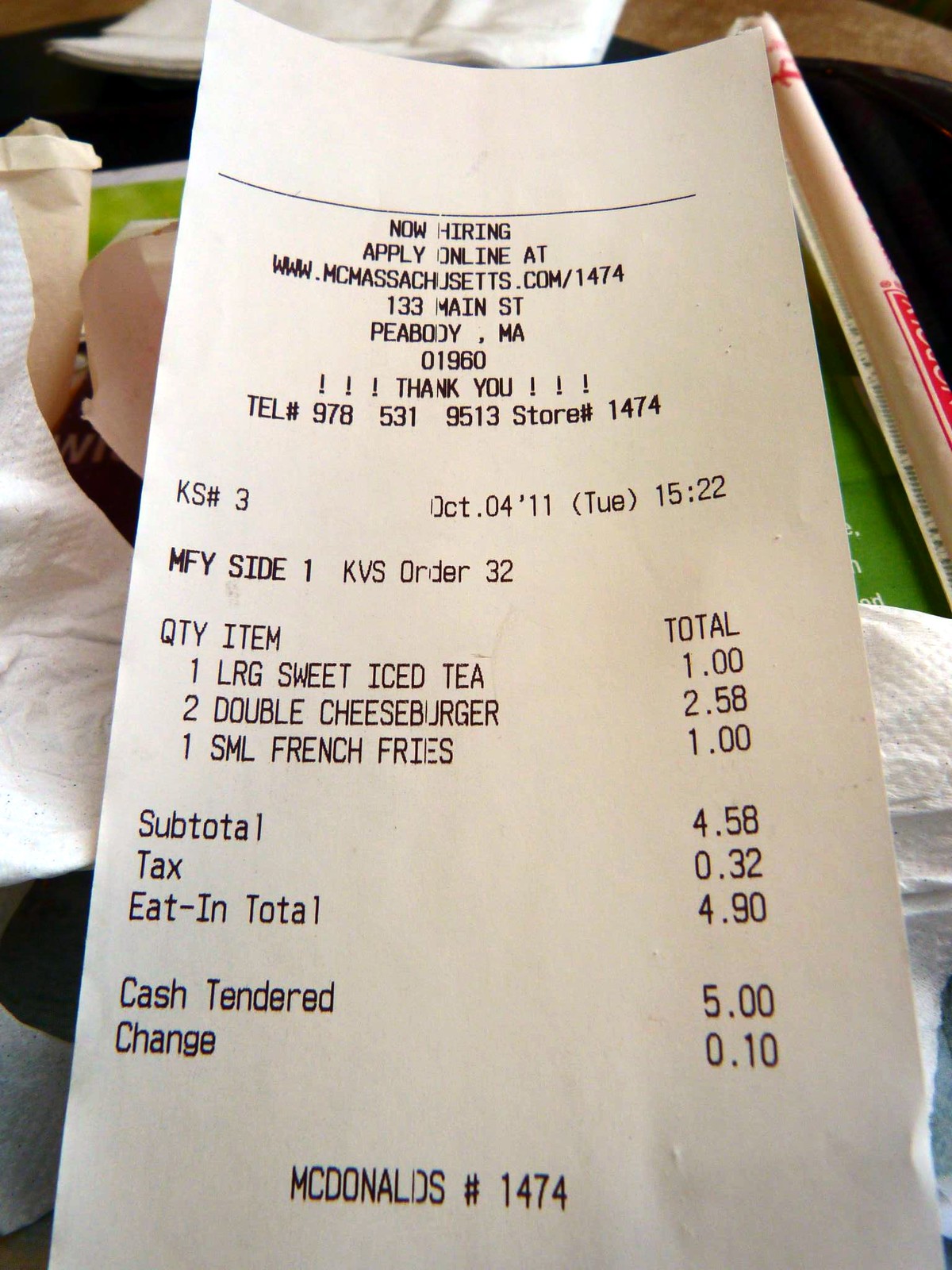This photograph captures an assortment of everyday items on a table. The main focus is on a white receipt printed in black ink, prominently displaying a message at the top that reads "Now Hiring, Apply Online." The receipt includes the address "133 Main Street, Peabody, Massachusetts, 01960" and thanks customers with a "Thank you" message. A phone number, "978-531-9513," and a store number, "1474," are also listed.

Beneath the receipt, partially visible, are some crumpled napkins and a red and white striped straw. There's also a small piece of green paper peeking out from underneath. The detailed transaction on the receipt indicates that the purchase was made on Tuesday, October 4, 2011, at 15:22. The items bought include one large sweet iced tea for $1.00, two double cheeseburgers totaling $2.58, and one small french fry for $1.00. The subtotal comes to $4.58 with an added tax of $0.32, making the total $4.90. The customer paid with a $5 bill, receiving $0.10 in change. The receipt also reiterates the McDonald's store number at the bottom.